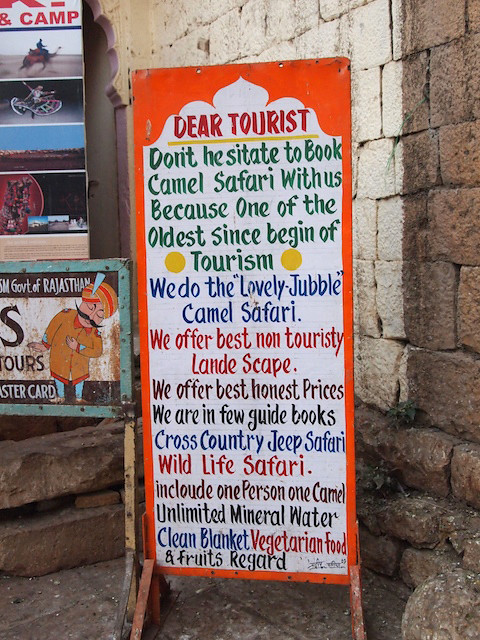This detailed photograph was taken outdoors, capturing the exterior of a potential tourist destination, possibly in India, the Middle East, or Africa. The focal point of the image is a large, vertically-oriented, rectangular orange metal sign, prominently placed in front of an old, brick wall. The vibrant sign, with a white background and text in various colors—red, green, blue, and black—starts with "Dear Tourist" in red font and provides a detailed offer for a Camel Safari experience. The text continues in green font, urging tourists not to hesitate to book with them as they are among the oldest providers since the beginning of tourism. It then describes a "lovely Jubble Camel Safari," boasts of offering the best non-touristy landscapes and honest prices, mentions appearances in a few guidebooks, and lists additional safari options such as Cross-Country Jeep Safari and Wildlife Safari, alternating the font colors among red, green, and blue for emphasis.

Included in the safari package is one person, one camel, unlimited mineral water, a clean blanket, vegetarian food, and fruits. To the left of this main sign, there are other smaller signs; one of these features images of a camel and possibly a bicycle, and another sign has the word "tours" with a graphic of a small man. The backdrop of cobblestones and the additional signage provide context to this enticing and colorful advertisement.